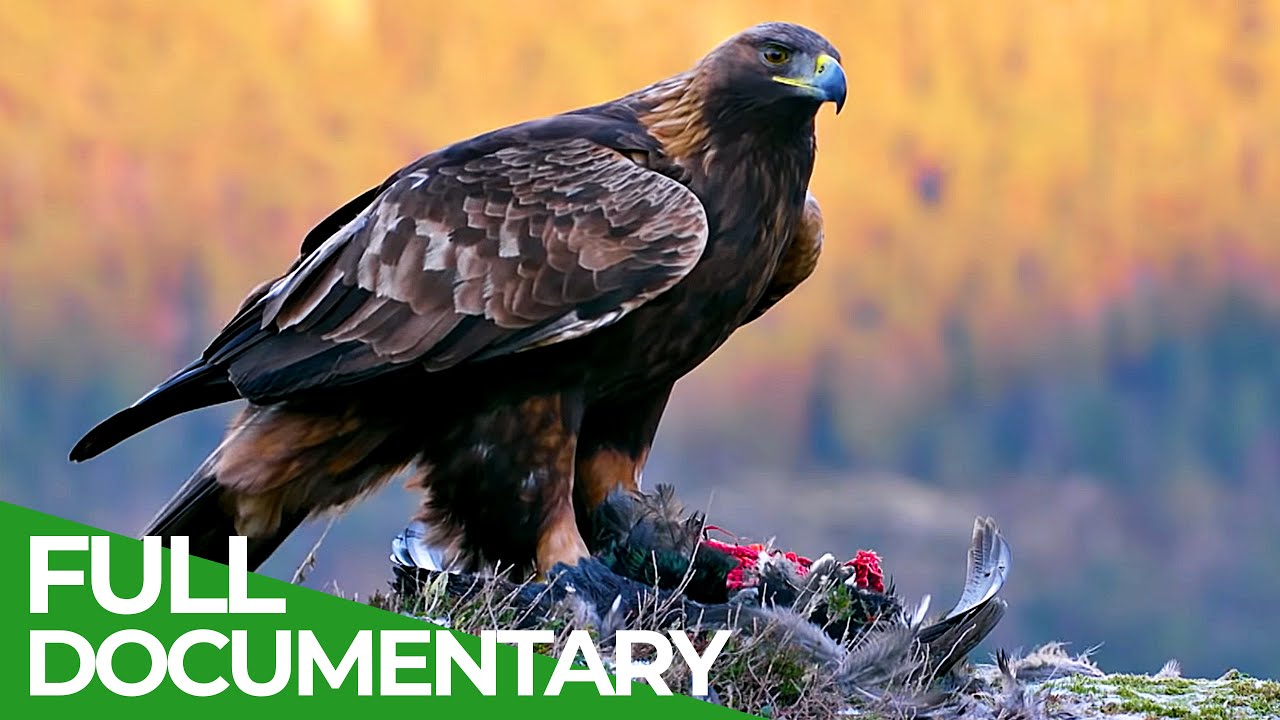This striking photograph, advertising a "Full Documentary," showcases a majestic bird of prey, likely an eagle, perched on a mound that appears to be the remains of another bird it has captured. The close-up reveals the bird's detailed features: a mix of dark black, brown, and gray feathers, with distinctive coloring on its wings. Its powerful beak is primarily blue, accented with yellow around the nostrils and mouth, and its piercing eyes gaze intently off to the right. The blurred forest backdrop, suggesting a colorful autumn setting, enhances the focus on the bird. The photograph includes a green triangle across the bottom, overlaid with the bold white text "Full Documentary," situated in the bottom left-hand corner.